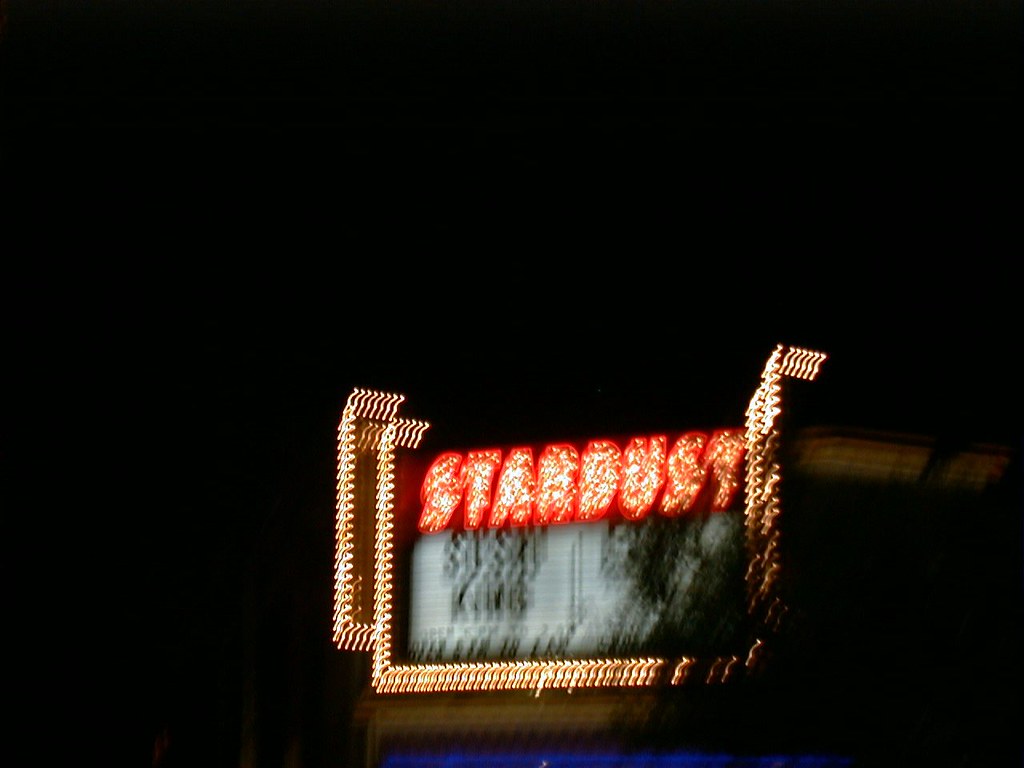This is a very blurry night-time photograph capturing an outdoor marquee affixed to a building. The marquee prominently features the word "Stardust" in a vibrant, yet slightly indistinct, display of bright red and orange-hued lights. These letters appear to be illuminated by yellow-orange light bulbs, with an outline likely created by red, possibly Xenon, bulbs. Beneath the "Stardust" signage, there's a section with letters on a white background, but due to their blurred and overlaid appearance, they remain unintelligible. The marquee is further framed by bright yellow lights along its borders. The overall image quality suggests it might be a close-up still from a video, which contributes to the difficulty in reading the text and the overall blurry nature of the photograph.